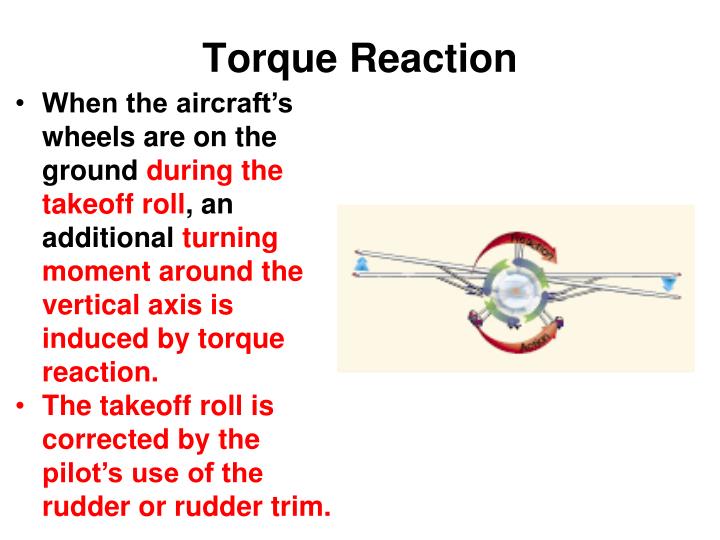The image titled "Torque Reaction" features a detailed description accompanied by a diagram. It consists of two bullet points with text in a mix of black and red colors. The first bullet, written mostly in black with phrases in red, explains that "when the aircraft's wheels are on the ground during the take-off roll, an additional turning moment around the vertical axis is induced by torque reaction." The second bullet, entirely in red text, states that "the take-off roll is corrected by the pilot's use of rudder or rudder trim." On the right side of the text, there is a diagram depicting an aircraft with wide wings. The diagram includes two red arrows indicating movement directions, set against a light pink background, while the rest of the image background is white.